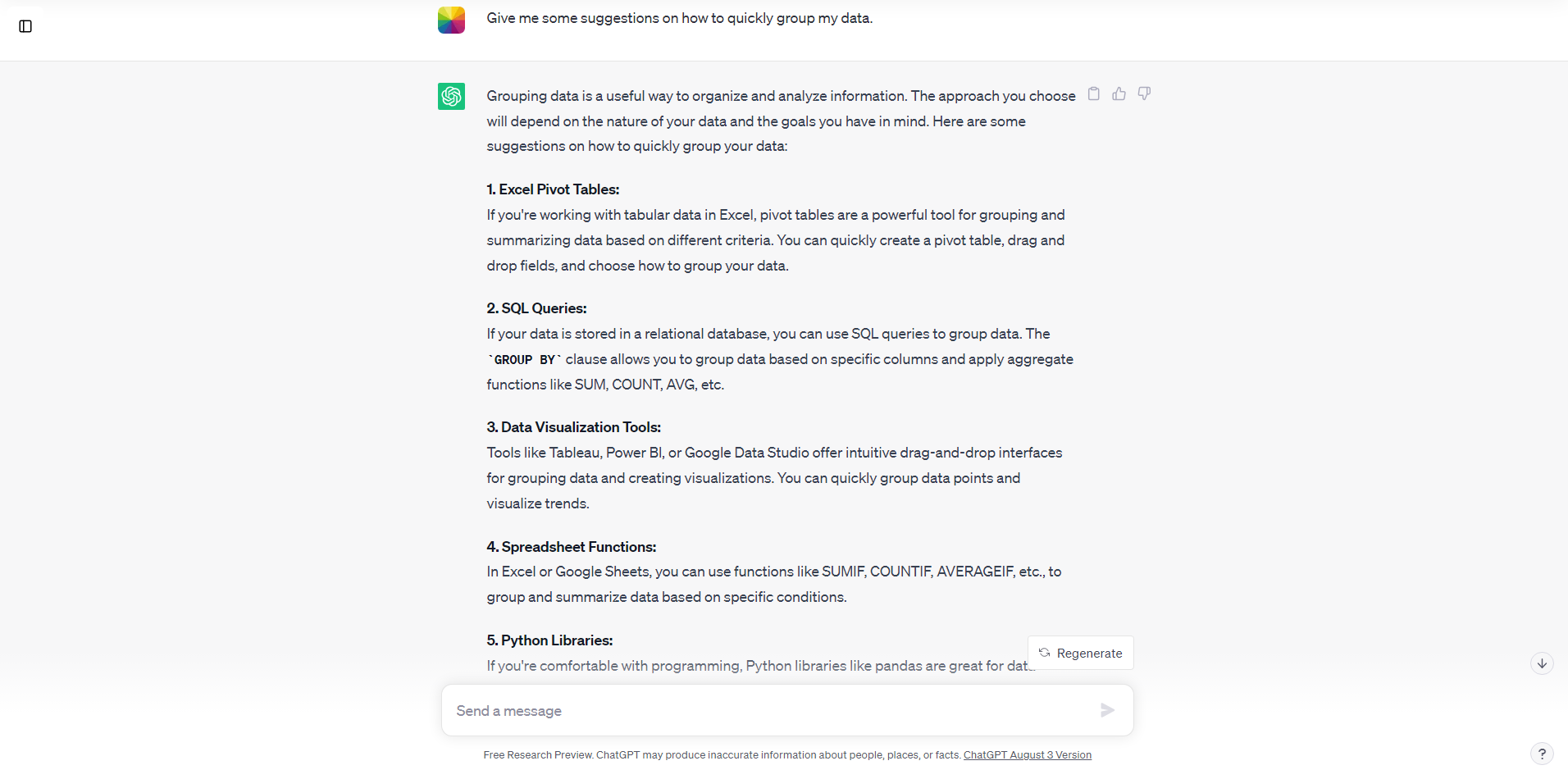**Detailed Caption:**

The image displays a helpful guide on quickly grouping data, set against a clean, visually appealing design featuring a white header and a light gray background. The guide emphasizes the importance of grouping data as an effective method for organizing and analyzing information, tailored to the nature of your data and your specific goals. It provides two main suggestions for grouping data:

1. **Excel Pivot Tables**: If you're working with tabular data in Excel, Pivot Tables are highlighted as a powerful tool for grouping and summarizing data based on different criteria. You can effortlessly create a Pivot Table, drag and drop fields, and select your preferred method for data grouping.

2. **SQL Queries**: For data stored in a relational database, the guide suggests using SQL queries to group data efficiently.

This structured, informative visual guide is designed to help users streamline their data organization process, catering to both spreadsheet and database environments.